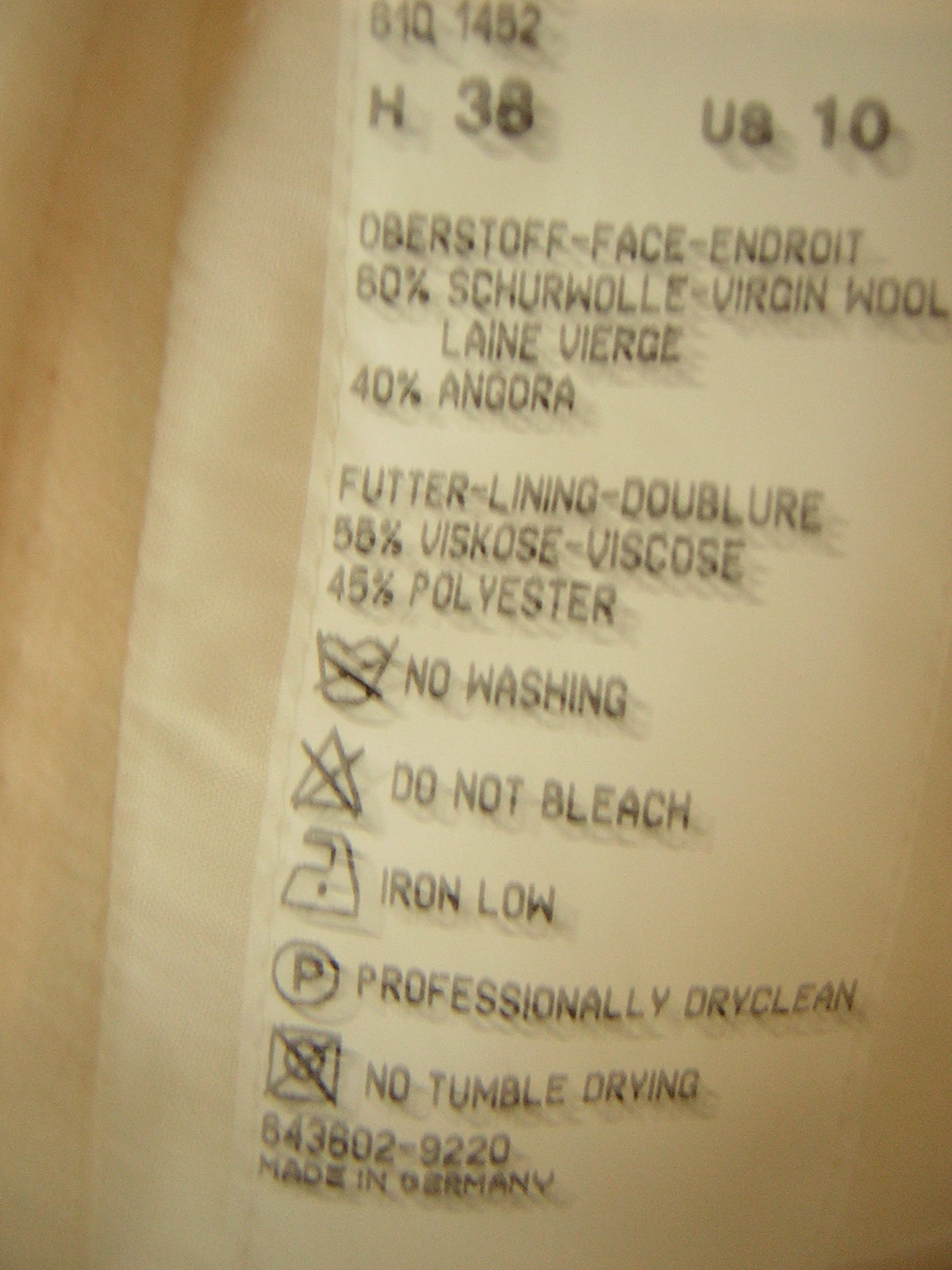This image features a detailed label against a light beige background, with a distinctive stripe of even lighter beige running through it. The top of the label displays a series of alphanumeric codes: "6 IQ 1452 h38 us-10." Below these codes, the label reads "Oberstdorf Face," followed by intricate product details in black text.

The label indicates that the material composition consists of 60% virgin wool and 40% angora. It also specifies the inner lining, which is made of 55% viscose and 45% polyester. The care instructions suggest no washing or bleaching, to iron on low heat, and to have the item professionally dry cleaned.